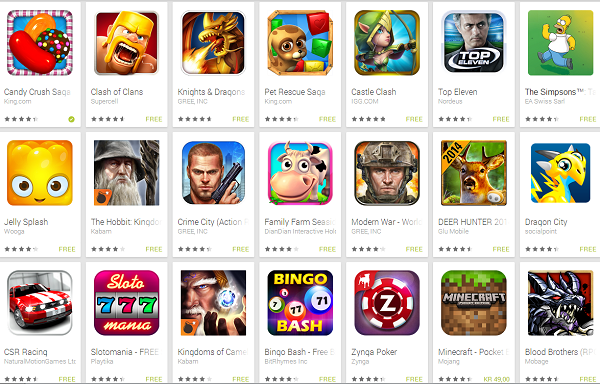This horizontal rectangular image features a neatly arranged grid of mobile app icons, divided into three rows, each containing seven icons. Below is a detailed description of each app icon from left to right:

**Row 1:**
1. **Candy Crush**: The icon showcases Candy Crush's signature design, featuring a candy cane border with a blue center, adorned with a red jelly bean atop an orange jelly bean, and a chocolate circle spruced with colorful dots.
2. **Clash of Clans**: This icon depicts a fierce-looking monster, emblematic of the popular strategy game.
3. **Knights and Dragons**: A dragon dominates the icon, breathing fire into the bottom-left corner of the image.
4. **Pet Rescue Saga**: The icon displays a cute little dog on a blue background, accompanied by colorful bricks to the right.
5. **Castle Clash**: An icon represents the game with its recognizable elements.
6. **Top Eleven**: The icon features a man with "Top Eleven" boldly written in white across the front.
7. **The Simpsons: Tapped Out**: It displays one of the iconic characters from the beloved TV series.

**Row 2:**
1. **Jelly Splash**: A charming, yellow jelly character graces this icon.
2. **The Hobbit: Kingdoms of Middle-earth**: While the last word is unreadable, the icon shows a man with a hat and a large, furry, cream-colored beard.
3. **Crime City**: The partial text "Action" is visible, with a man holding a gun aimed towards the upper right corner.
4. **Family Farm**: This icon features a friendly-looking cow.
5. **Modern War**: An army man is depicted in this icon, representing the military strategy game.
6. **Deer Hunter 2014**: A picture of a majestic deer with a small banner in the upper left corner indicating "2014."
7. **Dragon City**: A lively little yellow and turquoise dragon against a blue background.

**Row 3:**
1. **CSR Racing**: The icon shows a sleek red sports car with either gray or white stripes down the center, marking this popular racing game.
2. **Slotomania**: Featuring a slot machine with the word "slots" above and "Mania" below, displaying 777 in three different colors.
3. **Kingdoms of Camelot** (partial title): It pictures a man with bushy white eyebrows, a white beard, and mustache, holding a magical floating ball in his hands.
4. **Bingo Bash**: The text "Bingo Bash" is prominently displayed with four bingo balls showcasing numbers in the middle.
5. **Zynga Poker**: A poker chip with a "Z" in the center.
6. **Minecraft**: This icon includes the word "Minecraft" in gray font on a brown background, capped with green.
7. **Blood Brothers**: The icon showcases a monstrous character on a striking red background.

The image collectively captures the essence of popular mobile games and their distinctive icons.